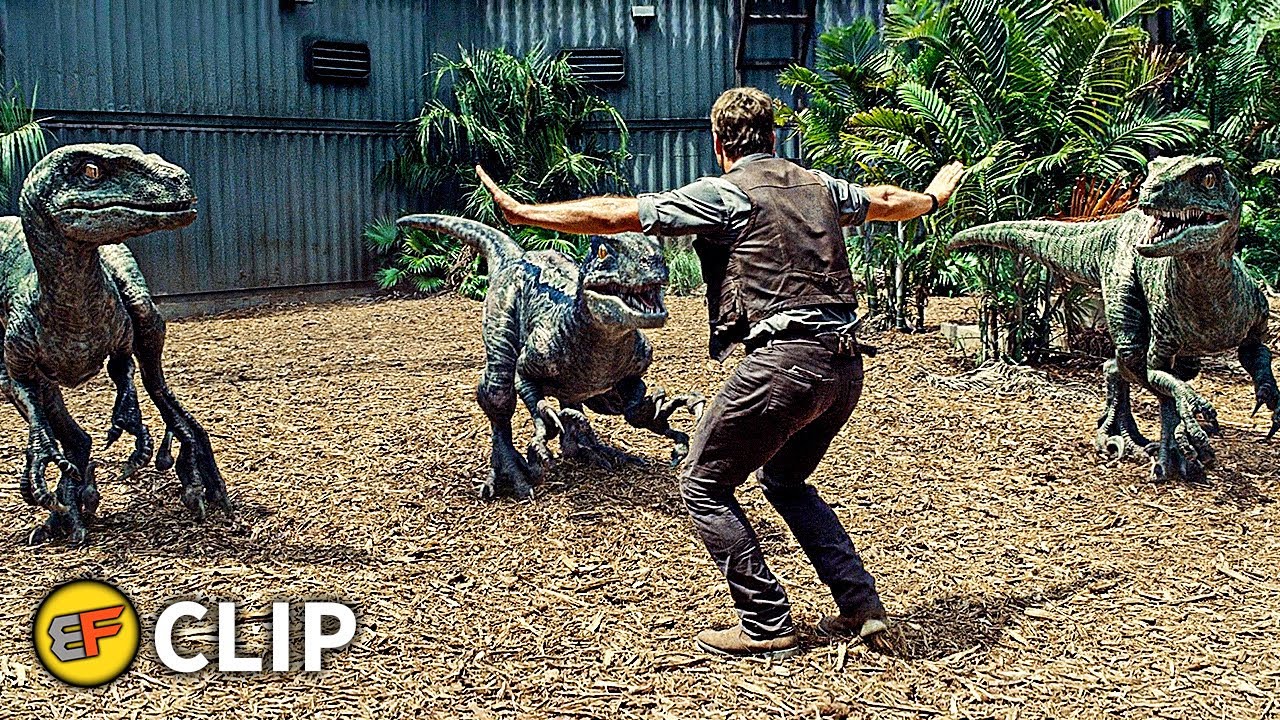In this screenshot from the movie "Jurassic World," a man, dressed in brown pants, light brown boots, a brown vest over a short-sleeved shirt, stands with his hands raised to his sides, attempting to control three gray, green-tinged velociraptors. The raptors, with their orange eyes, typical two large hind legs, two smaller forelimbs, and long tails, are positioned across the image — one on the left, one crouching in the middle, and one on the right, all focused intently on the man. The ground is covered in light-colored mulch or debris, and the scene is set in an enclosure bordered by a blue, aluminum-like shack building. Small plants and palm trees are visible around, with additional small palms to the right and one in front of the building. The image also features an EF clip indicator in the bottom left corner.